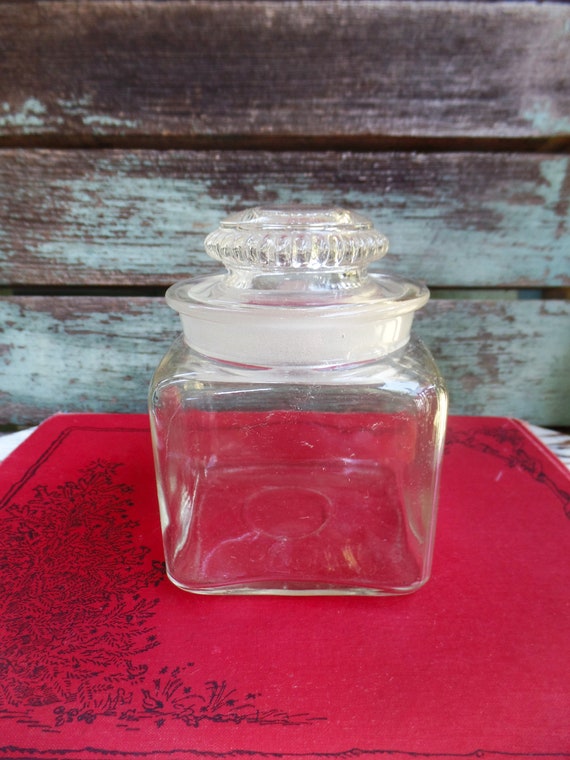In this photograph, a crystal-clear, square glass jar with a rounded top and a knob-like lid, decorated with cut-glass grooves, sits prominently on a red mat. This mat has a black border inset about an inch from the edges and features an intricate design of a bush with small black flowers in the lower left corner. The upper right corner of the mat has a small decorative cut that forms part of the border. The glass jar, which is designed to seal tightly with a rubber ring around the lid, is likely intended for storing candies. The scene is set on a wooden table or shelf, with worn, horizontal wooden slats in the background. These slats are faded to a light grey and brownish hue, giving the impression of an aged, possibly washed or weathered surface, like you'd see in an old, rustic house.